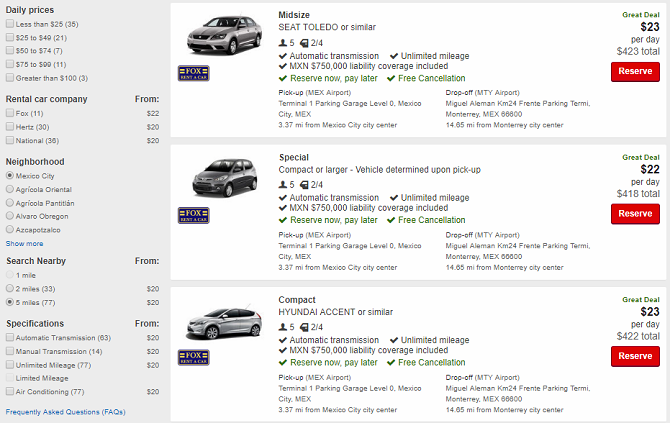The image features a detailed rental car booking interface. On the left side, a light gray sidebar displays various options in small text, including choices for daily prices, rental car companies, neighborhoods, search nearby, and specifications. Towards the top right section of the interface, there is an image of a gray car facing the camera but slightly angled to the left. The car is a midsize sedan described as "Toledo or similar," equipped with an automatic transmission, and offering unlimited mileage.

The booking details specify that the car rental includes MXN $750,000 in liability coverage. The pricing options highlight "Reserve Now, Pay Later" with conditions for free cancellation. The car can be picked up at Mexico City International Airport (MEX), Terminal One, Parking Garage Level Zero, which is approximately 3.37 miles from Mexico City's center. The drop-off location is Monterrey International Airport (MTY), Miguel Alemán KM 24, at the Frienday parking terminal in Monterrey, Mexico, with the postal code 66600.

Additionally, there's a green banner indicating that this rental is an excellent deal at just $23.